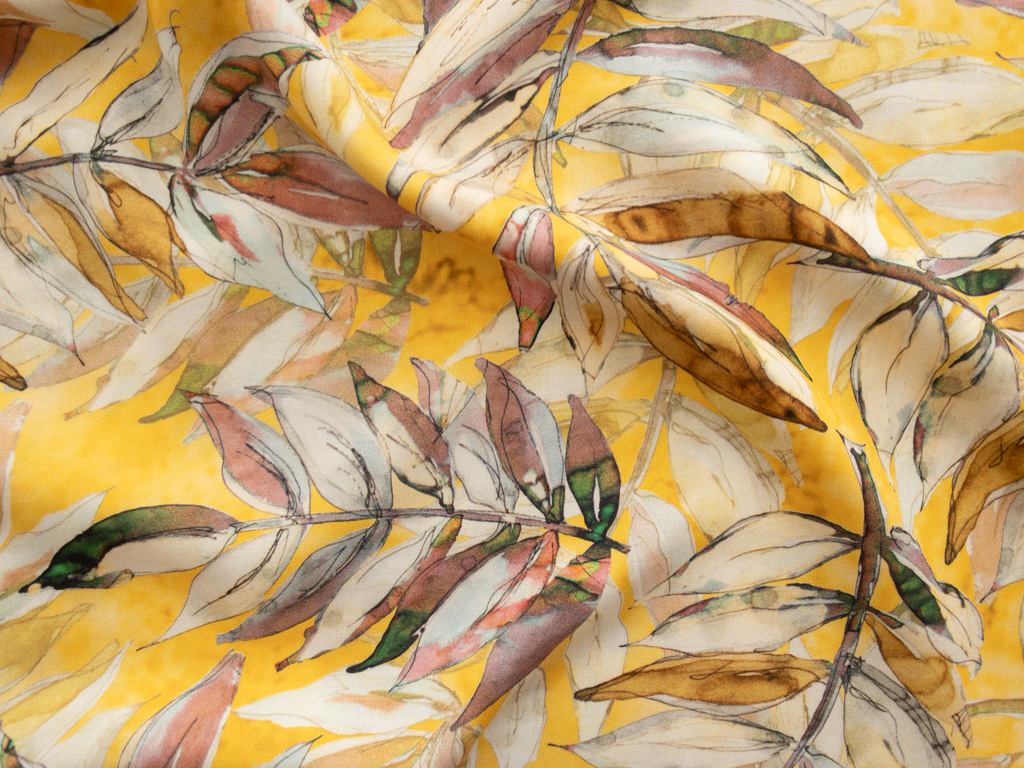The photograph captures an entire frame filled with a beautifully draped piece of yellow fabric characterized by smooth, rounded creases. The fabric has a bright, yet slightly mottled yellow background, providing a striking backdrop for the painted leaves that adorn it. These leaves, rendered in a loose, abstract watercolor style, are arranged in delicate branches with approximately 13 leaves each, positioned oppositely along the stems. The leaves display a colorful palette of white, pink, green, pale yellow, and golden hues, creating a vibrant and whimsical floral pattern. The branches and leaves overlap and extend in various directions, contributing to an airy, wispy appearance. The fabric extends beyond the edges of the photograph, enclosing the entire visual space and enhancing the textured elegance of the scene.